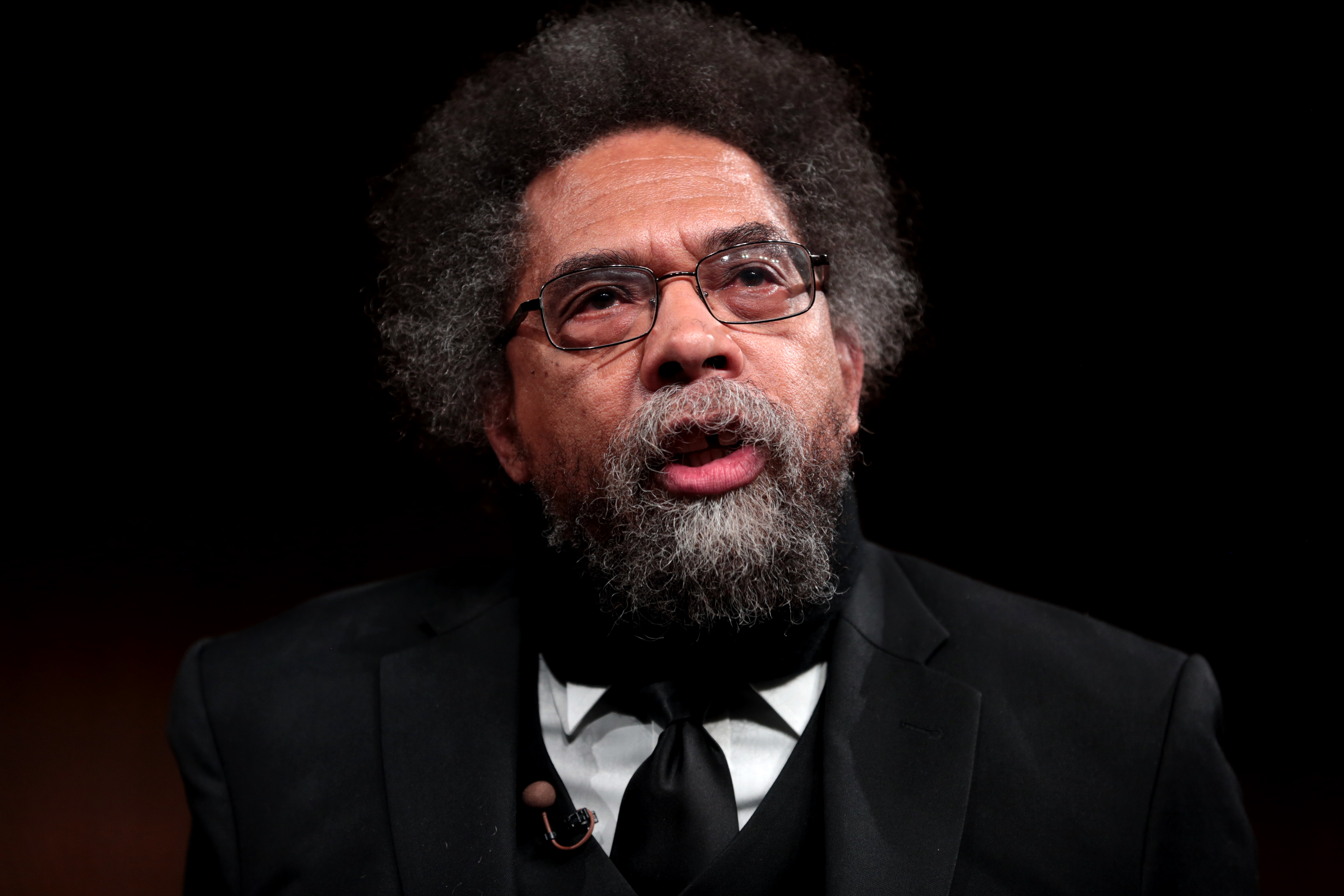An older Caucasian man with frizzy black and grey hair, complemented by a matching beard and moustache, is the subject of this photograph. He is adorned in small, black-framed glasses that sit above dark-colored eyes. His mouth is slightly open, presenting a glimpse into a moment of speech, though the darkness of the image obscures his teeth. Clad in a black suit jacket with a white shirt and a tightly knotted black tie, he exudes a formal demeanor. A small brown microphone is clipped to the left side of his suit jacket, indicating he might be addressing an audience or participating in an interview. Against a completely black background, the edges of his attire blend seamlessly, emphasizing the solitary and introspective nature of the scene.